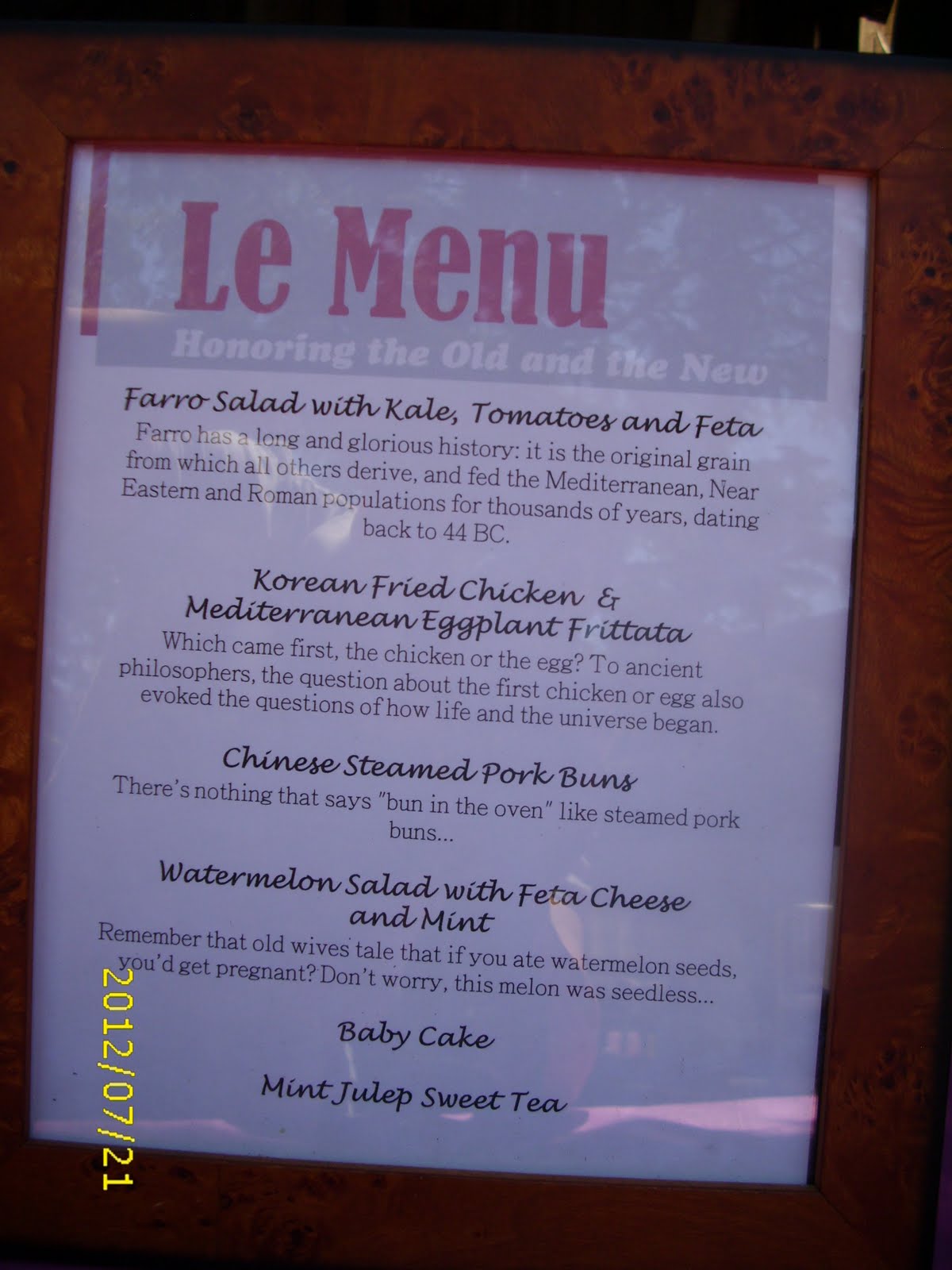In this detailed image, we see a single white menu page placed on a dark brown wooden table. The menu has a subtle red border at the top and prominently displays the title "Le Menu" in large red letters. Just beneath this, in elegant white lettering, is the phrase "Honoring the Old and the New," framed by a barely noticeable, almost transparent decorative border that evokes the imagery of trees and the sky.

The menu entries are meticulously detailed, beginning with "Faro Salad with Kale, Tomatoes, and Feta" in black text. A succinct history of faro follows in smaller letters, noting its ancient origins and significance: "Faro has a long and glorious history. It is the original grain from which all others derived and fed the Mediterranean, Near Eastern and Roman populations for thousands of years, dating back to 44 B.C."

Next, in bold text, are the offerings "Korean Fried Chicken and Mediterranean Eggplant Frittata," accompanied by an intriguing philosophical note: "Which came first, the chicken or the egg? To ancient philosophers, the question about the first chicken or egg also evoked the questions of how life in the universe began."

Following this, "Chinese Steamed Pork Buns" is presented in black bold letters, with a whimsical remark in smaller letters: "There's nothing like this that says bun in the oven, like steamed pork buns..."

The subsequent item, "Watermelon Salad with Feta Cheese and Mint," is again highlighted in bold, with a small amusing anecdote: "Remember the old wife's tale that if you ate watermelon seeds, you'd get pregnant? Don't worry, this melon was seedless..."

The dessert offerings are simply listed as "Baby Cake" and "Mint Julep Sweet Tea," both in larger bold black letters.

Lastly, vertically aligned on the left side of the menu page in yellow text is the date "2012/07/21," adding a subtle yet interesting historical context to the menu.